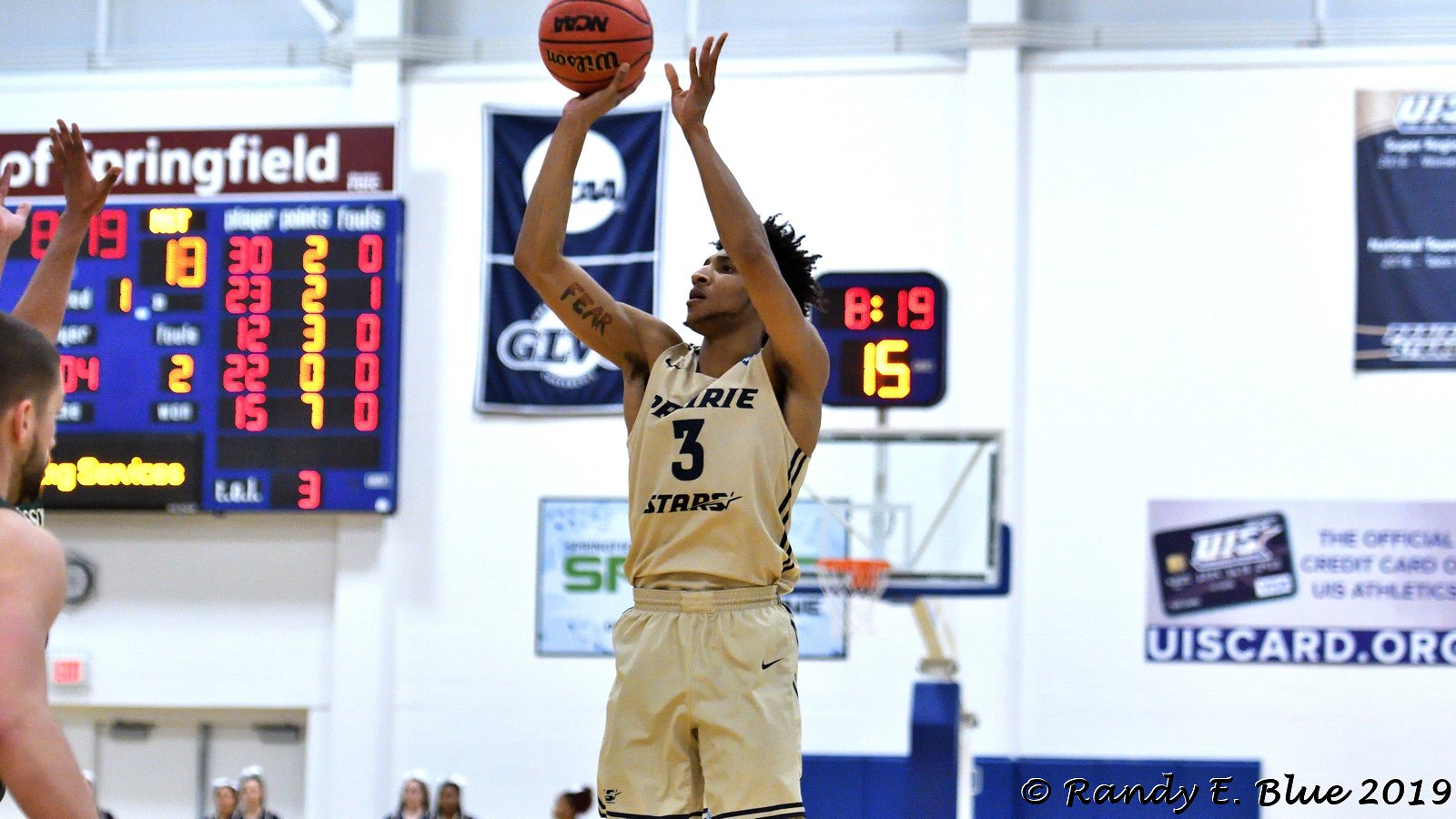In this detailed photograph captured inside a school basketball arena, a male basketball player with spiky hair, wearing a Nike-made cream-colored uniform with navy blue stripes and the number 3 on his jersey, is seen in midair as he attempts a shot, likely a three-pointer. The ball is held in his right hand, while his other hand is also raised. His uniform prominently features the word "Stars" and he sports a visible tattoo on the inside of his upper right arm that reads "fear." The background showcases an indoor gymnasium with white walls, a partially visible basketball hoop, and multiple posters advertising various items. Behind the jumping player, a scoreboard reads 8 minutes and 19 seconds and shows a score of 15. On the other side, another scoreboard, partly legible, displays the word "Springfield" and indicates two fouls. Seen around the lower edge of the photograph are the heads of several spectators and the out-of-focus forms of a couple of cheerleaders with hair bows. A white male defender, positioned approximately two feet in front of the shooting player, has his arm raised, attempting to block the shot.